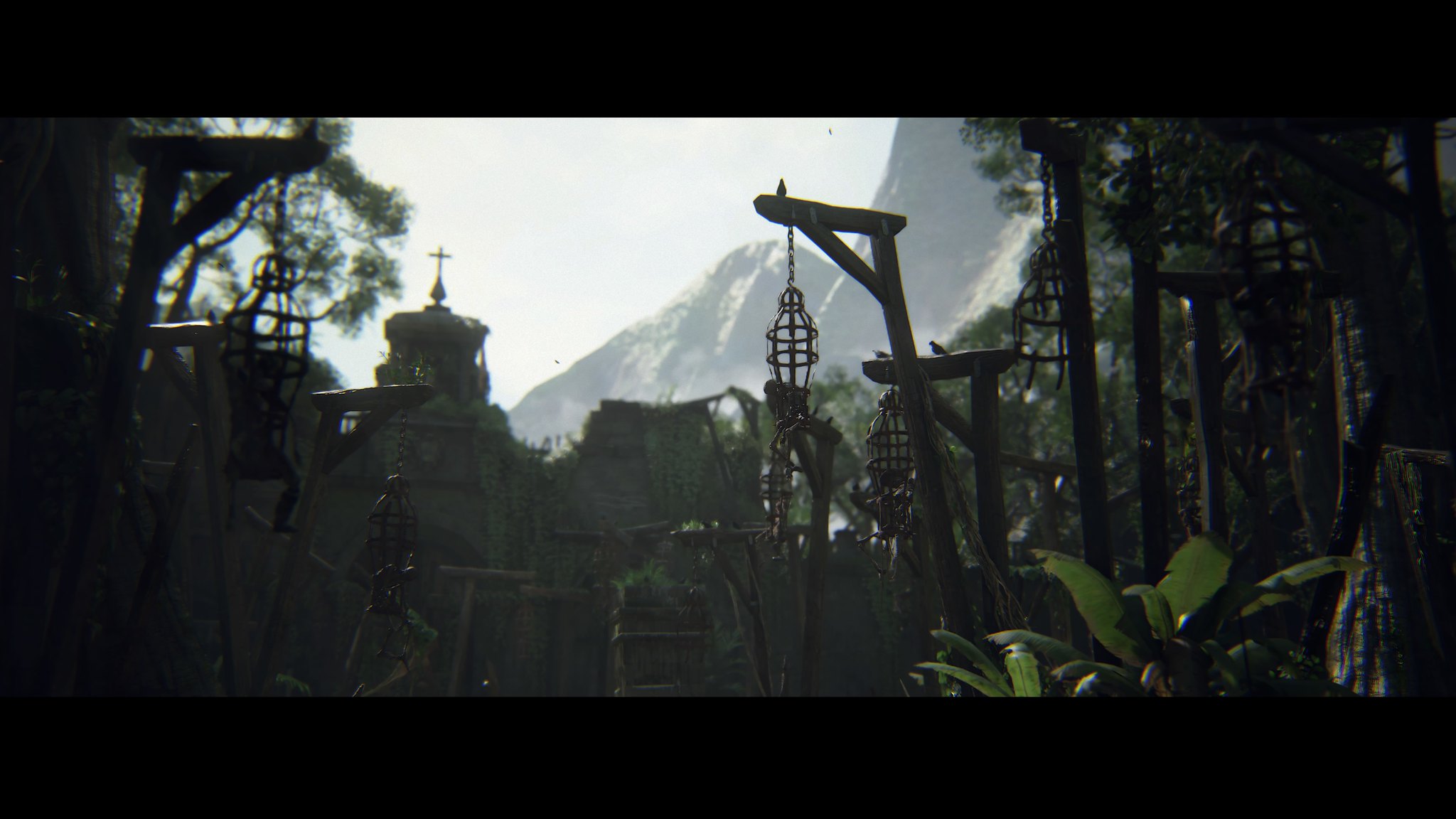The image depicts six cage-like lanterns, each adorned with various hanging objects. In the background, a towering mountain dominates the scene under a bright, white daytime sky. Centrally positioned to the left, a cross symbol stands prominently on top of a large ledge, suggesting a location of religious significance. The top corners of the image are framed by tree branches and leaves, adding depth and natural beauty. In the bottom right corner, a plant with large green leaves further enhances the picturesque setting. The overall atmosphere suggests that this might be the site of an ancient church or a historical religious landmark.